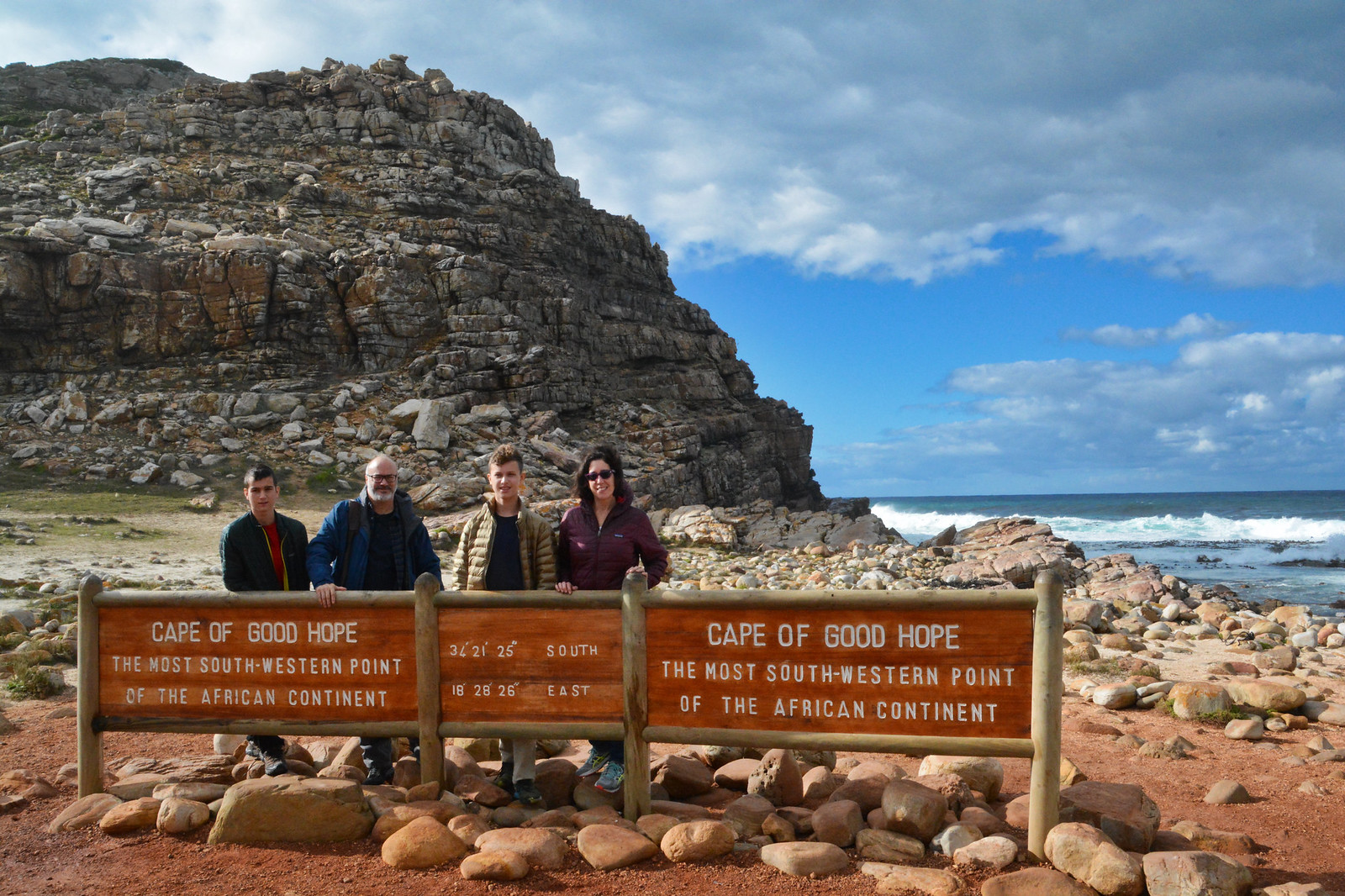In this vibrant travel photo, four individuals, likely a family, are captured standing on a rocky beach at the Cape of Good Hope, the most southwestern point of the African continent. Behind them, the scene is dominated by a rugged, jagged rock mountain with the vast ocean and a partly cloudy blue sky stretching into the horizon. The family is positioned behind a red wooden sign arranged as a triptych. The left and right sections of the sign announce "Cape of Good Hope, the most southwestern point of the African continent," while the middle section provides the precise coordinates: 34° 21' 25" S, 18° 28' 26" E.

From left to right, the people in the photograph include a man in a light spring black coat over a red shirt, an older balding man with white hair, glasses, and a blue coat over a blue shirt, a young man donning a gold puffy jacket with a black shirt, and a black-haired woman wearing sunglasses and a purple shirt. They stand among the scattered rocks, genuinely embodying the adventurous, tourist spirit at this famous landmark.